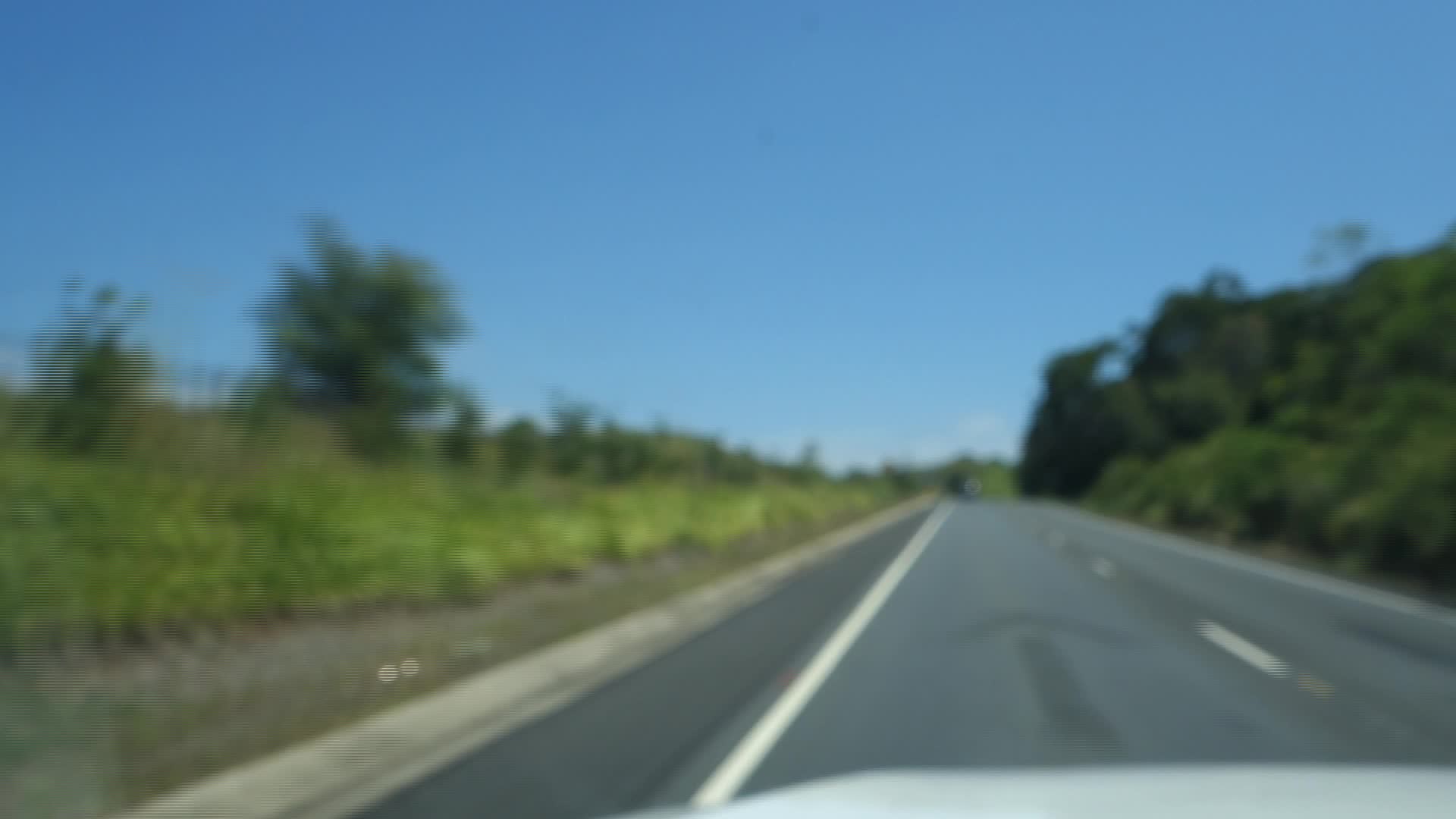This is a photograph taken from the front windshield of a car on a blurry, sunlit country highway. The scene features a two-lane asphalt road running diagonally from the bottom right towards the upper left of the frame. Both lanes head away from the viewer, with a faded directional arrow barely visible on the lighter gray pavement. The road is bordered by a solid white line on the left and a dashed white line in the center.

To the right of the roadway, there's a bike lane paved in darker asphalt, and beyond that, a sidewalk leading up to some greenery. This side of the road is lined with low bushes and taller, dark green trees. On the left side, lighter green vegetation and grassy patches can be seen, along with a possible cement curb. The sky, occupying about half of the image, is a clear, bright blue, void of clouds, indicating a clear day. The entire photograph, though detailed in scenery, remains out-of-focus, giving it a somewhat indistinct appearance.